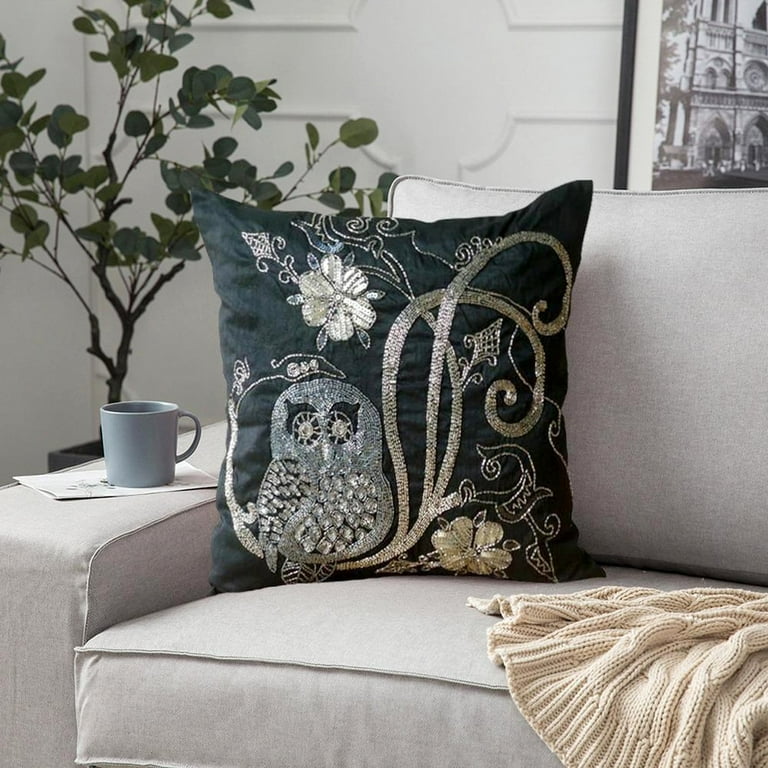This image captures a meticulously designed living space with an emphasis on a decorative couch pillow. The pillow, positioned near the arm of a gray couch, features a detailed design showcasing a light blue and white owl perched on a branch, with additional motifs such as a white flower and possibly some vines. To the right of the owl, there's a gold flower detail. The pillow's artwork is intricate, reminiscent of Art Nouveau style.

The gray couch is accented with a cream-colored throw blanket draped over it. On the arm of the couch, a light blue coffee mug rests atop a greeting card or pamphlet. Behind this setup, a small green plant in a barely visible pot adds a touch of nature to the scene.

In the background, a textured wall with relief patterns serves as an elegant backdrop. A framed black and white artwork, possibly depicting a European-style cathedral like Notre Dame, hangs prominently on the right. The room's cohesive color palette and carefully chosen decor elements highlight the work of a skilled interior designer.